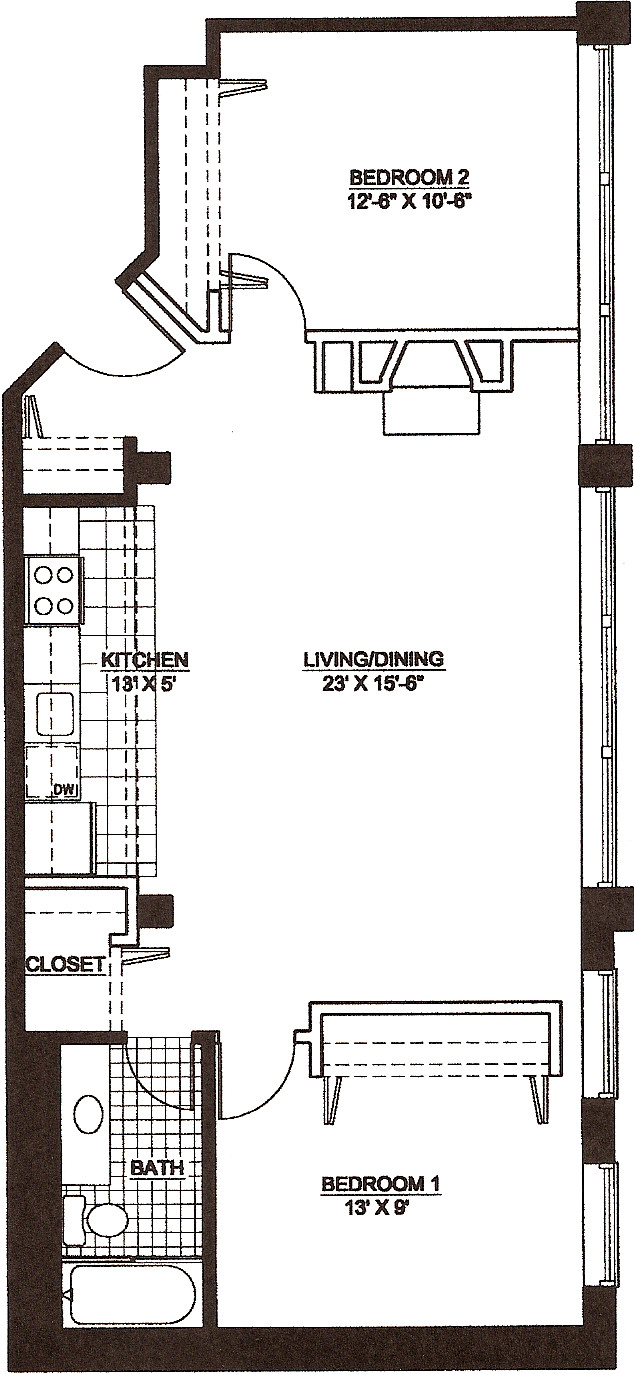Detailed Architectural Drawing Caption: 

This architectural drawing presents a detailed layout of a specific section of a home, arranged in a vertical orientation. The bottom portion features a rectangular form that narrows towards the top. At the top of the drawing, "Bedroom 2" is prominently labeled in black letters on a white background, with dimensions specified as 12 feet 6 inches by 10 feet 6 inches. Below this, the layout transitions into a spacious living and dining room area, also demarcated in fine black lines and annotated with dimensions of 23 feet by 15 feet 6 inches.

Further down the layout, "Bedroom 1" is detailed as occupying a space of 13 feet by 9 feet. Adjacent to Bedroom 1, on its left, a bathroom is illustrated, equipped with a tub, a toilet, and a vanity with an integrated sink. Above the bathroom layout, a closet space is designated. Both bedrooms are outlined with door placements, and each bedroom has a narrow, elongated closet.

To the left of the living and dining area, the kitchen is delineated, marked with dimensions of 13 feet by 5 feet. The kitchen floor is denoted with tile symbols and includes detailed drawings of the various fixtures: a sink area, a stove with four burners, a dishwasher labeled "DW," and a larger box assumed to be a refrigerator. This drawing provides a comprehensive and precise representation of the designated home section, highlighting key spatial dimensions and room functionalities.